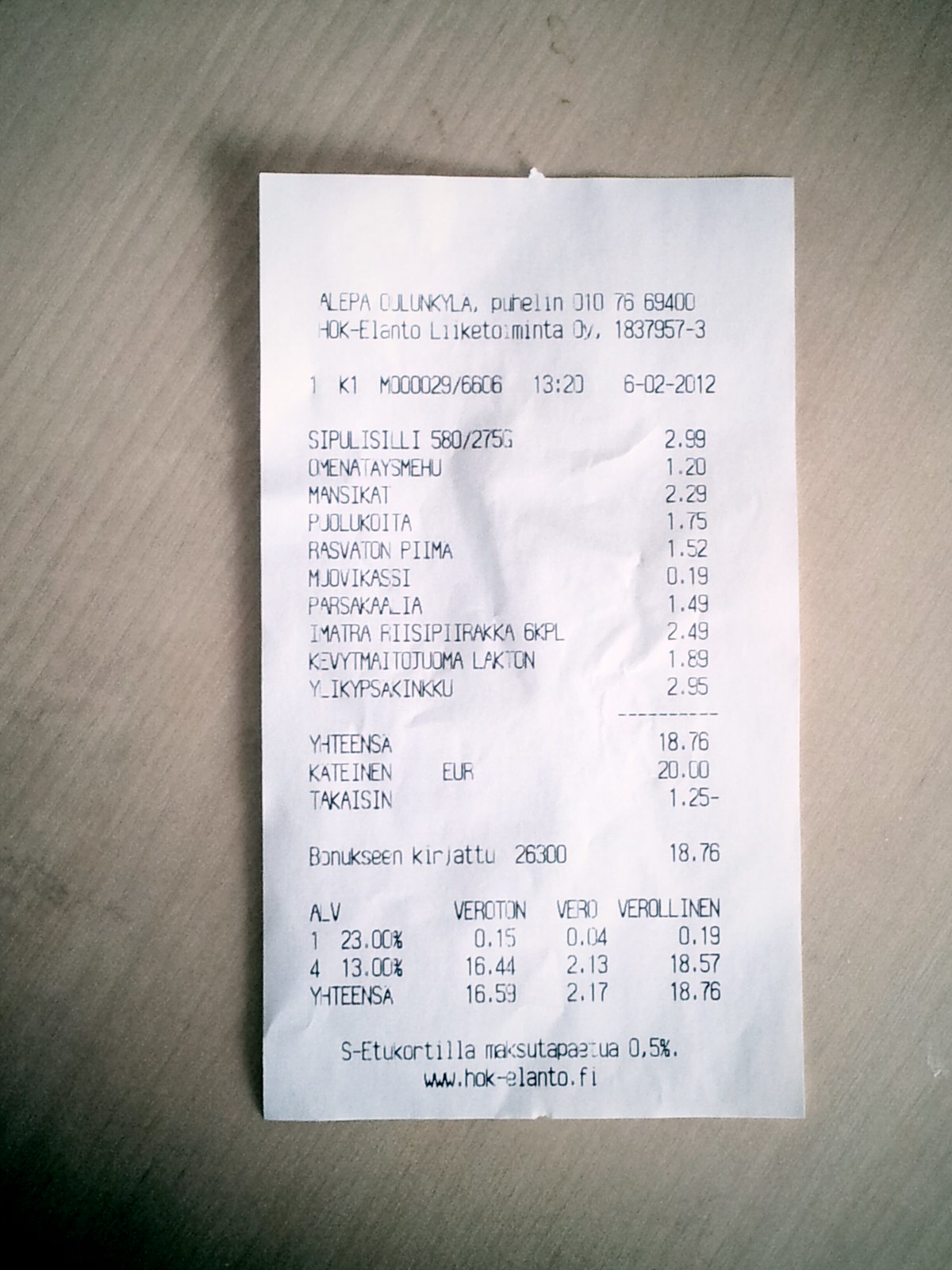The image is a color photograph of a white receipt laying on a beige wooden table with noticeable vertical grain lines slanting to the right. The receipt, printed in a foreign language presumed to be Finnish due to the website www.hok-elanto.fi at the bottom, details a grocery purchase. The itemized list features food items left-aligned, with corresponding prices right-aligned. At the top, the store's name and address are visible, followed by the purchase date of 6-2-2012 at 13:20. The receipt documents the purchase of ten different items, culminating in a total of $18.76. The customer paid with a $20 bill and received $1.25 in change.